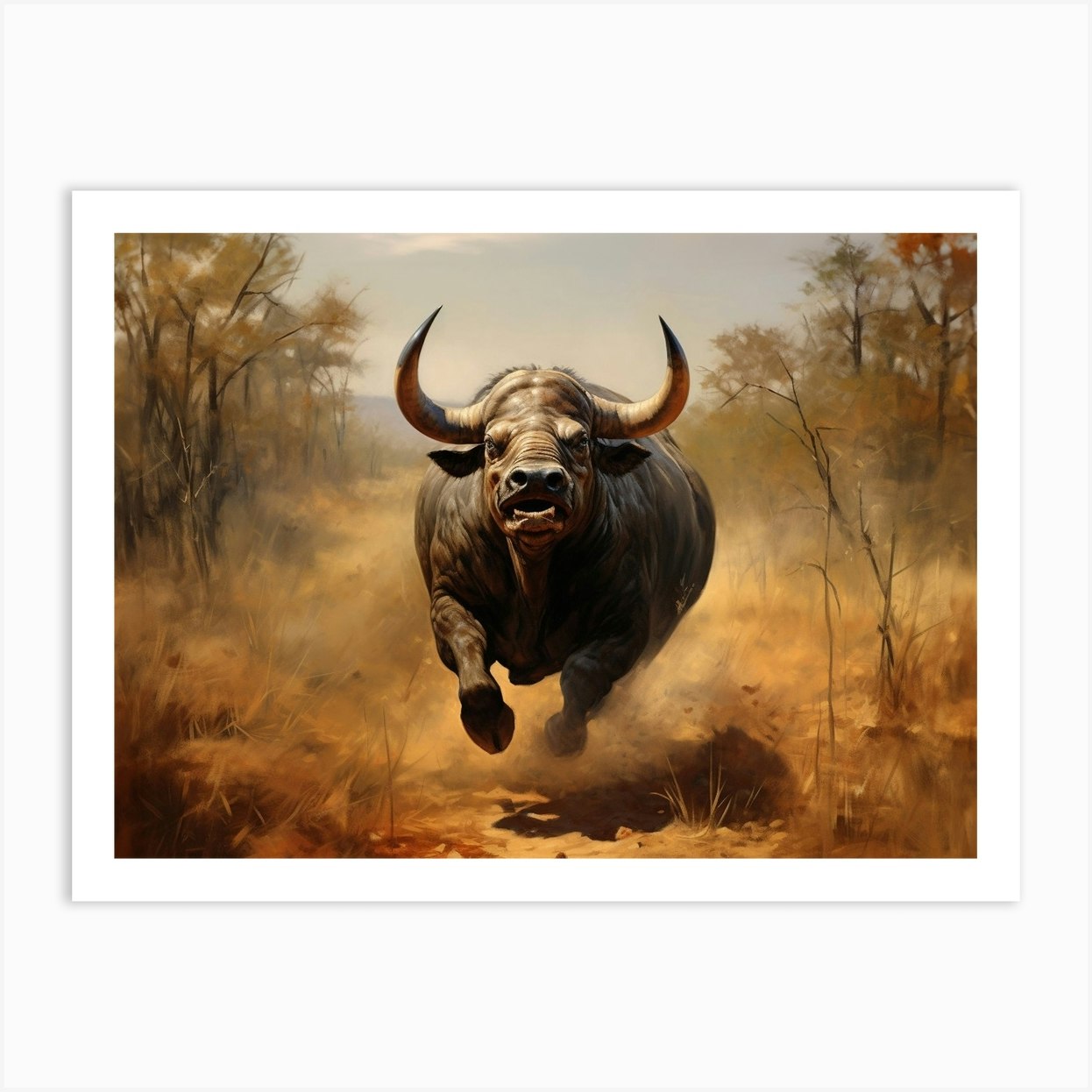This hyper-realistic painting captures an enormous, dark brown bull charging directly towards the viewer with vigorous energy and anger. Its powerful body, resembling a blend of a bison and a rhino, kicks up a cloud of dust and dirt as its front hooves lift off the ground in mid-gallop. The bull's large, upward-pointing horns frame its head, while its mouth is slightly open, revealing its bottom teeth, and its eyes are intensely focused. The scene is set in a dried, earthy landscape, with brown and tan grass, sparse vegetation, and bare tree branches on both sides, all under a blue sky dotted with a few wispy clouds. The entire piece is bordered by a white frame, suggesting it's a photograph or postcard depiction. Shadows under the bull and the detailed texture of its wrinkly skin enhance the realism, making it appear as though the beast is about to break through the image.